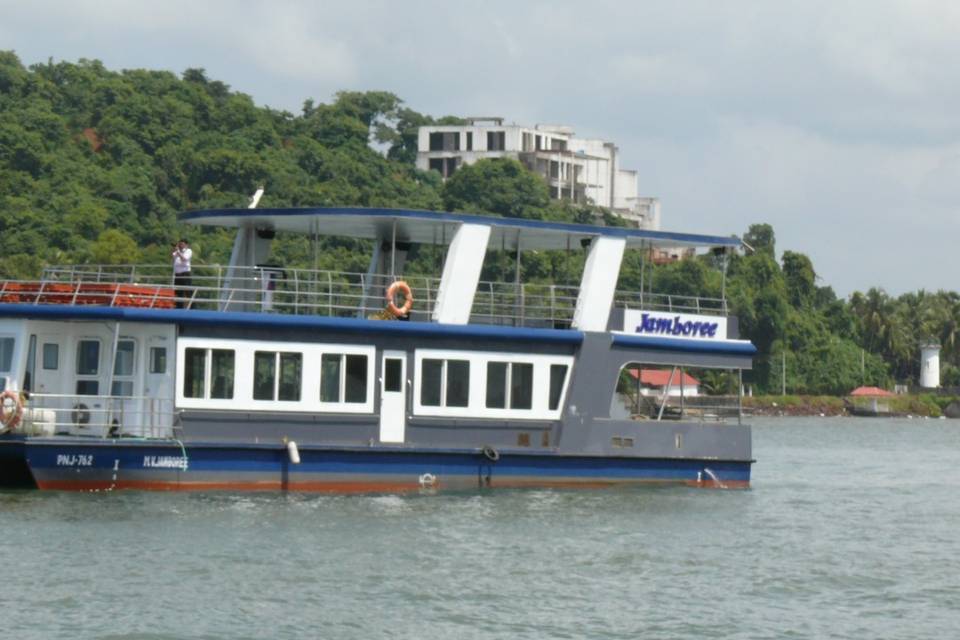This image captures a double-decker boat named "Jamboree" navigating on a body of water, slightly off-center to the left. At the bottom of the image, the water exhibits ripples, indicating a gentle breeze. The boat serves a dual purpose, potentially as a party or tourist vessel. The lower deck is enclosed with numerous windows and a rear open deck, while the upper level is open and surrounded by metal railings, featuring a covered top for passengers to stroll and enjoy the view. An orange life buoy hangs on the top railing. The upper level also has a visible man standing towards the front. In the backdrop, a verdant hill adorned with various trees rises, crowned by a sizeable white multi-level building, which could be an apartment complex or office building. Additional smaller structures with red roofs, including a potential gazebo and a lighthouse-like object, dot the shoreline. The setting conveys a warm, tropical ambiance.